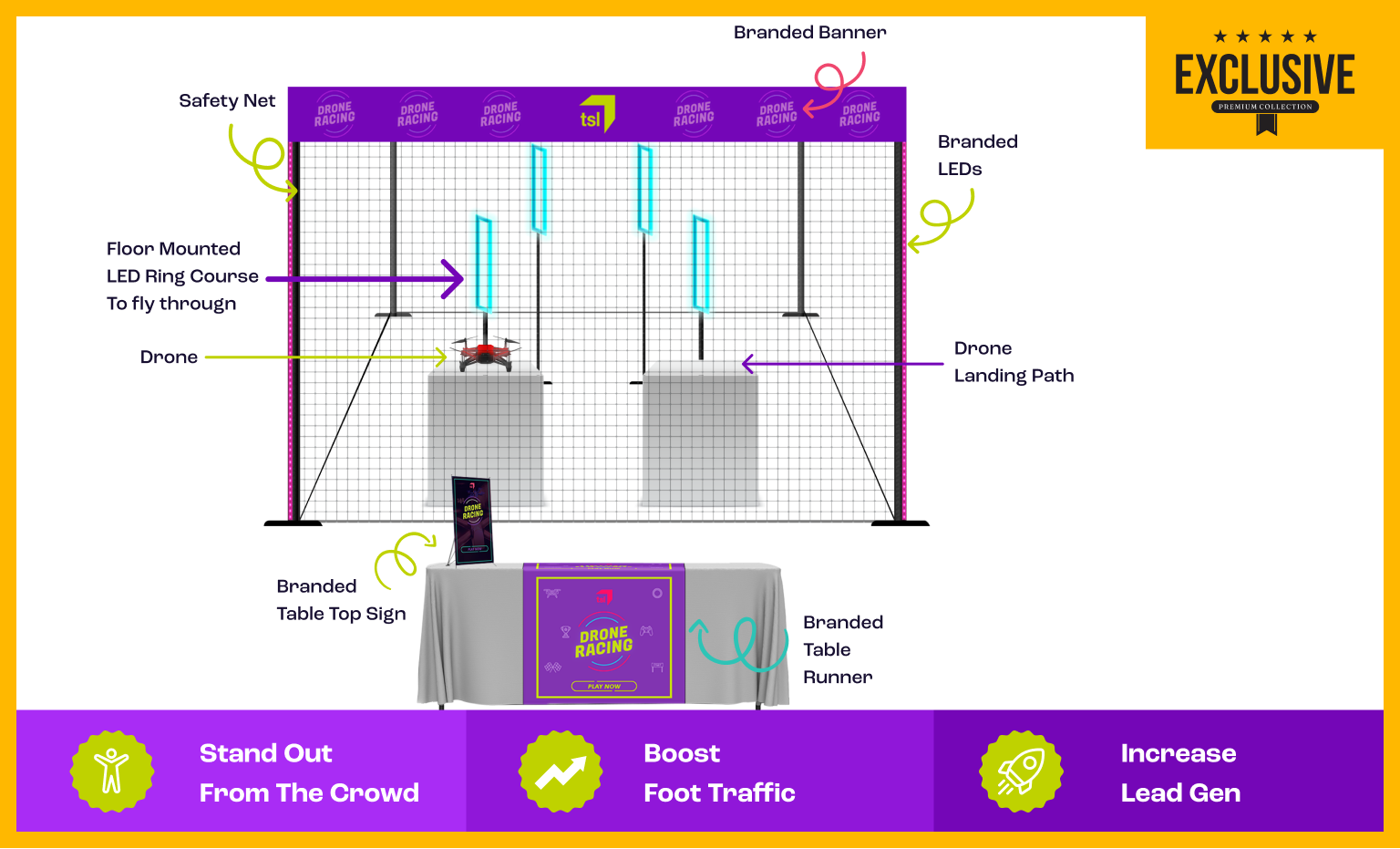The image serves as an advertisement for an exclusive, premium collection focused on drone racing, highlighted by a diagram showcasing the setup of a trade show booth aimed at grabbing attention and boosting engagement. In the top right corner, framed by a yellowed border that dips into the page, is a highlighted box featuring five stars and the words "Exclusive Premium Collection." 

The central diagram details a floor-mounted LED ring course with a red drone navigating from table to table, each outfitted with branded elements such as tabletop signs and table runners. The surrounding environment, including components like a drone landing pad on another table and a safety net, suggests that the setup is meant to be demonstrated within a contained, cage-like structure.

The design is vibrant, featuring a primarily white background accented with bold golds, purples, lime greens, and a touch of blue. Three prominent purple blocks at the bottom emphasize the key benefits of this setup: "Stand out from the crowd," "Boost foot traffic," and "Increase lead generation." These details, combined with branded LEDs and strategic placement of promotional materials, illustrate how this arrangement can elevate your presence at a trade show or similar event.